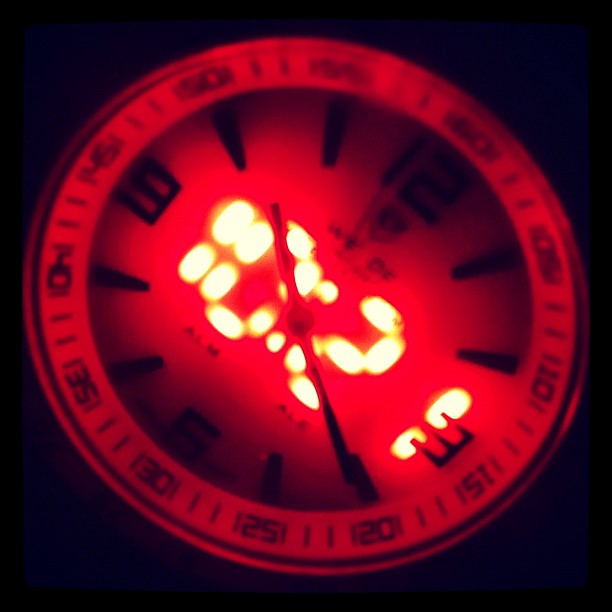This photograph captures a watch face glowing vividly against a pitch-black background, emphasizing its striking red illumination. The face of the watch is both digital and analog. At the center, red digital numbers display the time, reading 10:21, which is echoed by the position of the analog hands—the hour hand pointing to 10 and the minute hand to 4. Surrounding this, the watch face features only the cardinal numbers 12, 3, 6, and 9, while intermediary dials are marked with incremental intervals of 5 units up to 60. The watch's circular border also emits a red glow, enhancing its visibility in the dark. The entire setting underscores a scene taken at night, with the stark contrast between the glowing red elements and the surrounding blackness adding a dramatic effect.